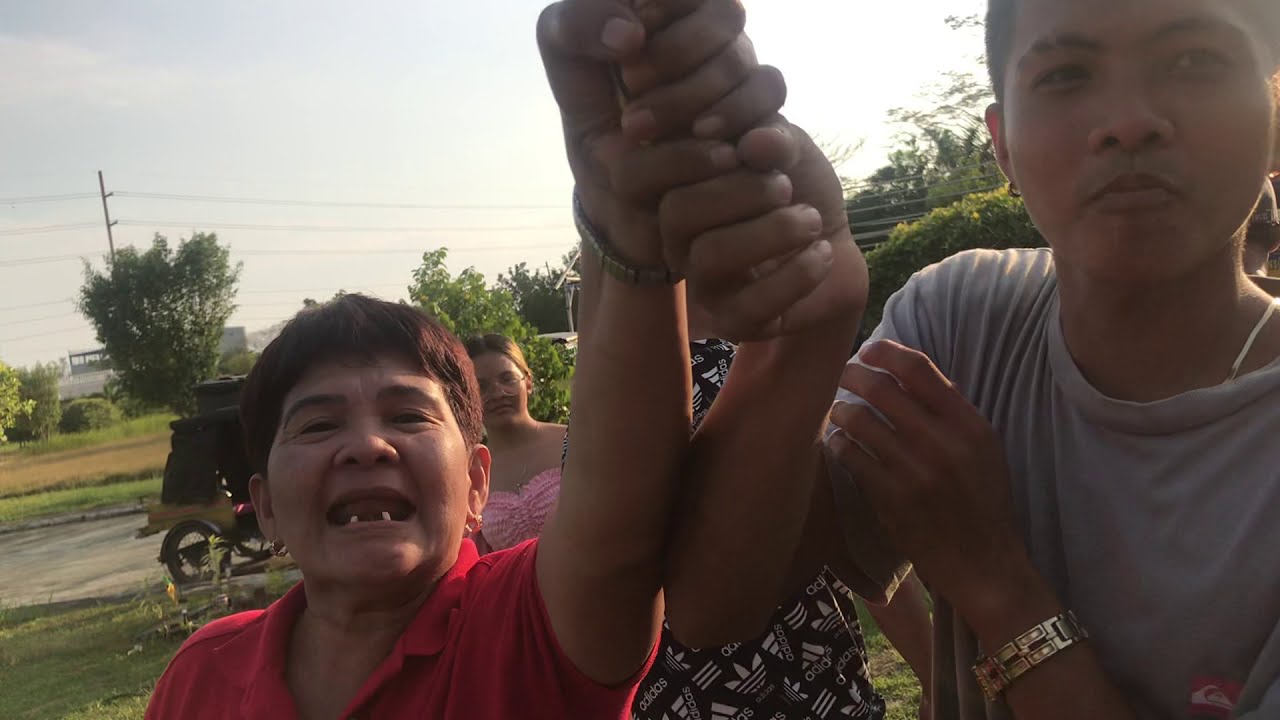This outdoor photograph captures a moment involving several individuals, likely of South Asian descent, standing under a bright, sunny sky. At the center is a young boy in his early twenties, sporting a light gray short-sleeved t-shirt and a gold bracelet. He holds hands with an older woman in her late 70s, clad in a short-sleeved red t-shirt, who appears happy with a gummy smile, only two bottom teeth visible. Their hands are raised high, and they are accompanied by another figure whose face is obscured, wearing a black Adidas shirt emblazoned with white logos.

To the side and slightly behind them stands a younger girl, perhaps a teenager, dressed in a sleeveless light pink top and glasses. She watches the central figures with interest. The background is rich with detail, featuring power lines, trees, and a mixture of buildings and what looks like a factory. A motorcycle cart bike and some wheels, presumably part of a vehicle, are also visible, adding to the rural, open-road feel of the scene surrounded by greenery.